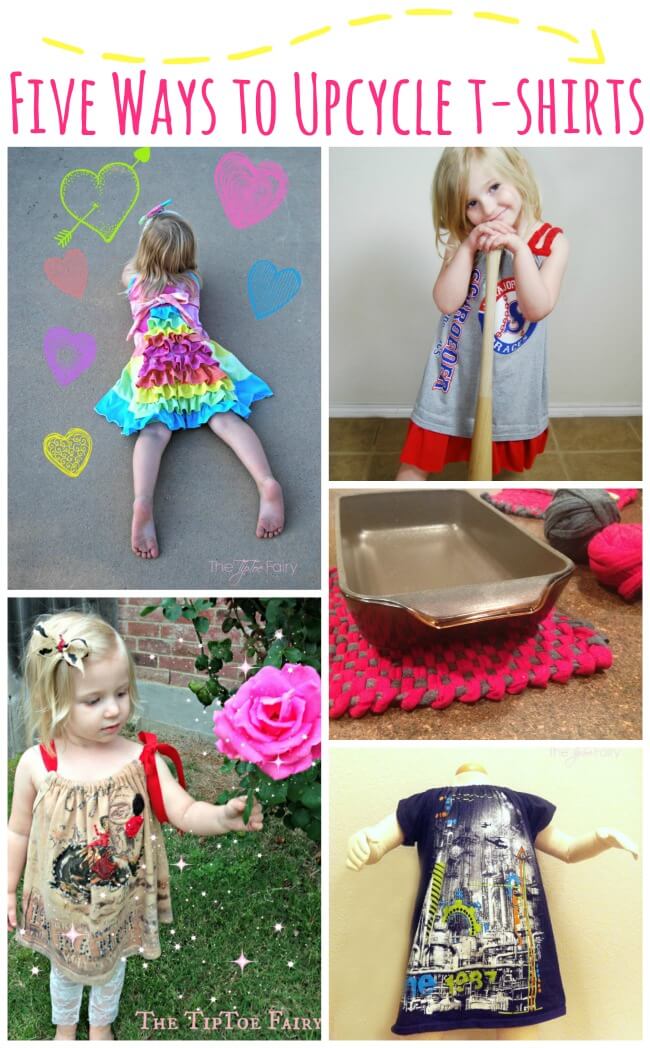The image features a white background with the bold, fuchsia pink title "Five Ways to Upcycle T-Shirts" at the top, accompanied by a decorative yellow squiggle line pointing right. Below this, the image is divided into five sections, each showcasing different creative ideas for repurposing old t-shirts. 

The first section on the left depicts a young girl lying on her stomach on a sidewalk surrounded by chalk-drawn hearts. She is wearing a vibrant, rainbow-colored ruffle dress, presumably made from upcycled t-shirts. To the right, in the second section, the same girl leans her chin on a baseball bat, smiling and dressed in a two-layered gray and red outfit featuring a baseball design, also a product of t-shirt upcycling.

The third section showcases a bronze-colored baking pan resting on a bright pink potholder, suggesting an alternative use of old t-shirts as kitchen accessories. In the fourth section, a headless mannequin displays a navy blue shirt with an abstract white and blue design, likely a cityscape, demonstrating how t-shirts can be transformed into stylish apparel.

Finally, the fifth section on the left shows the same girl outdoors, reaching for a pink rose in a garden while wearing a sundress with colorful straps and accompanying leggings, another example of t-shirt transformation. Each segment collectively illustrates inventive and visually appealing ways to give old t-shirts new life.